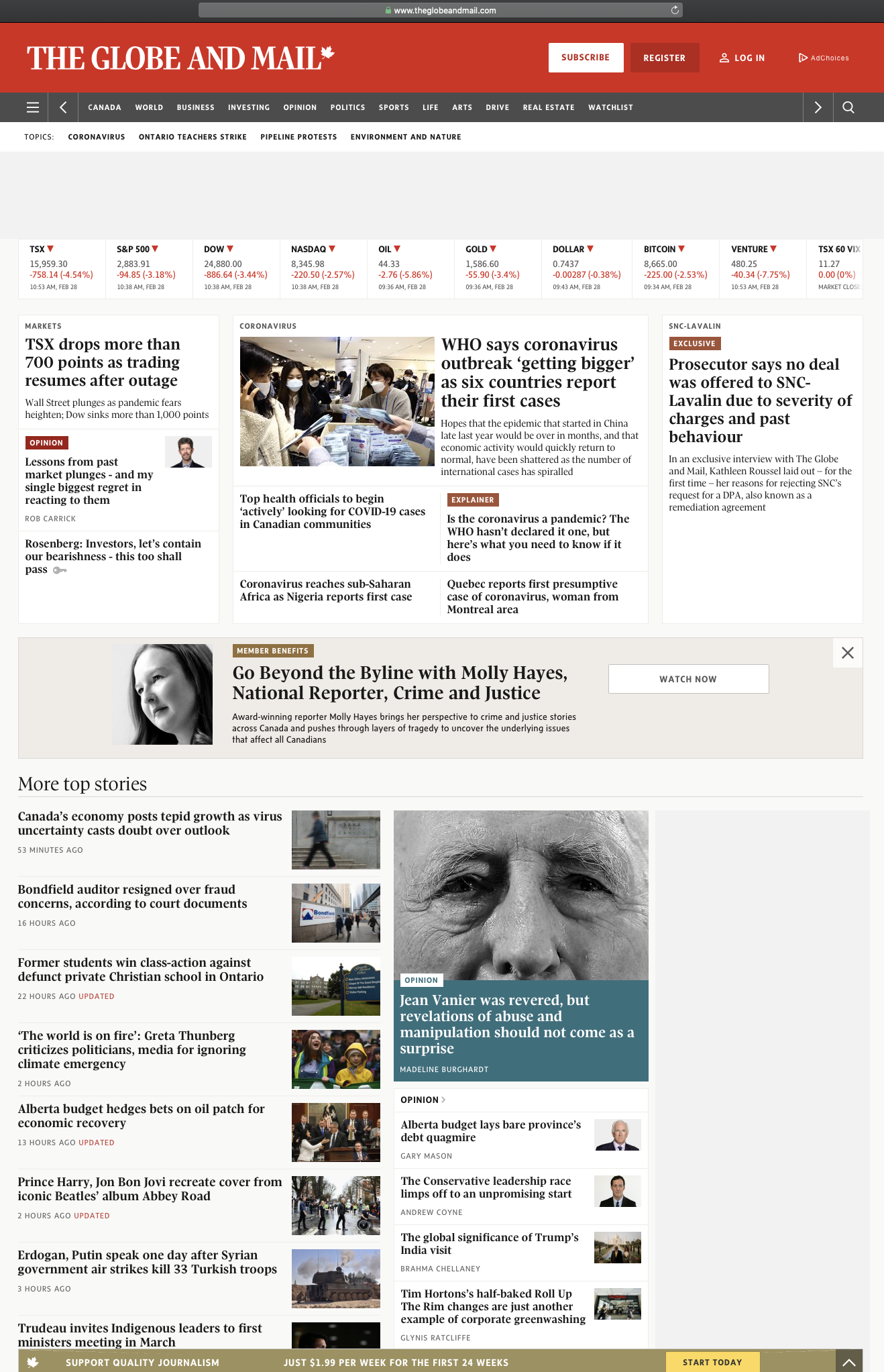At the top of the image, there is a thick red border with the title "THE GLOBE AND MAIL" in bold white capital letters, alongside a Canadian maple leaf icon angled to the right. Below it, a white rectangle features the word "SUBSCRIBE" in red lettering. To its right, a maroon rectangle reads "REGISTER" in white text. Further right, "LOG IN" appears in white letters next to a small outline of a person, followed by the recognizable AdSense by Google logo featuring a right-pointing triangle.

Beneath this header, a dark grey menu bar is displayed, containing three horizontal lines symbolizing a drop-down menu. Adjacent to it, a left-pointing arrow suggests a back option. The menu bar lists categories including: "Canada," "World," "Business," "Investing," "Opinion," "Politics," "Sport," "Life," "Art," "Drive," "Real Estate," and "Watchlist." An arrow pointing to the right and a search icon conclude the menu bar.

Further down, a series of black menu options highlights topics such as: "Coronavirus," "Ontario Teachers Strike," "Pipeline Protests," and "Employment & Environment." Additionally, stock market figures are presented in a sequence of black and light grey text, interspersed with red and light grey lines.

In the upper middle left portion, a prominent headline reads: "TSX drops more than 700 points as trading resumes after outage." To its right, another headline states: "WHO says coronavirus outbreak getting bigger as six countries report their first cases." Further right, a third headline declares: "Prosecutors say no deal was offered to SNC-Lavalin due to severity of charges and past behavior."